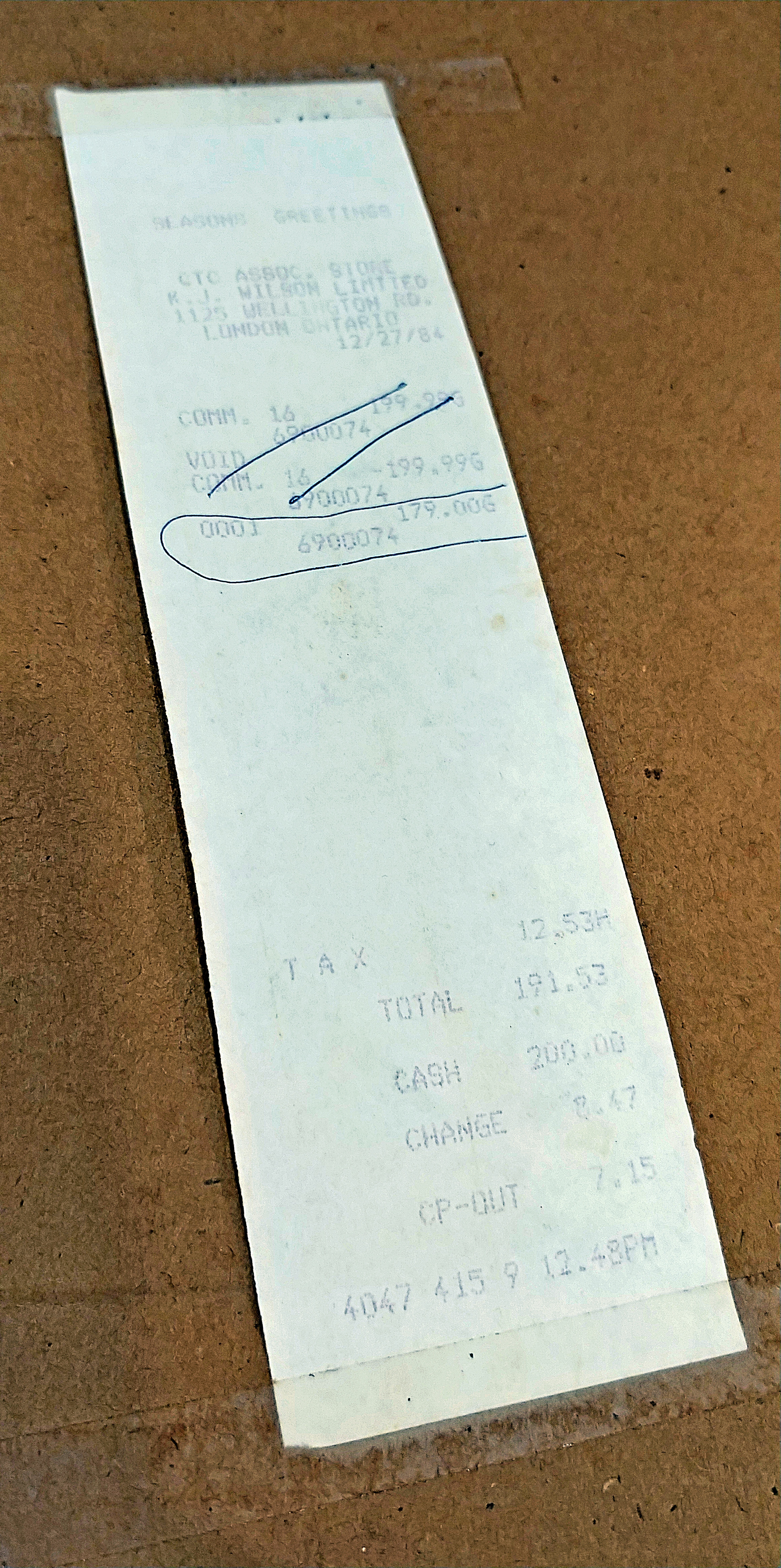This is a detailed color photograph of a long, white receipt placed on a dark brown surface. The top of the receipt features the text "Seasons Greetings." Below this, there is some writing that is too blurry to decipher. Further down, it reads "London, Ontario 12/27/84." A section of the receipt has been crossed out with blue ballpoint pen, and another section is circled, displaying the numbers "0001179.00 G 6900074." Towards the bottom, the receipt lists the tax amount as "12.53 H" and the total as "193.53." It then shows a cash payment of "200" and a cash balance of "8.47." Additional text includes "CP - out 7.154 047 415 912," and the time stamped is "4:48 p.m." The receipt appears to be affixed to the brown surface with clear scotch tape.